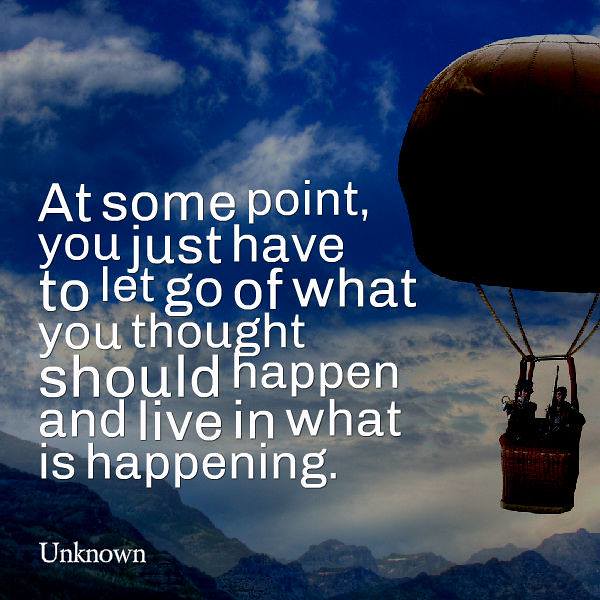The image is a vertical, rectangular motivational poster featuring a scenic view of the sky and mountains. The backdrop showcases a predominantly blue sky adorned with wispy white clouds, some of which almost appear blue. The lower portion of the image reveals distant mountains with a few snow-capped peaks. On the right side of the image floats a hot air balloon, shrouded in shadows that obscure its exact color, though it appears beige. The balloon has a brown basket holding two figures who resemble old-timey individuals, possibly one wearing a top hat.

The serene and picturesque setting is complemented by a motivational quote placed on the left side of the image. The text, written in white, reads: "At some point, you just have to let go of what you thought should happen and live in what is happening." The quote is attributed to "Unknown."